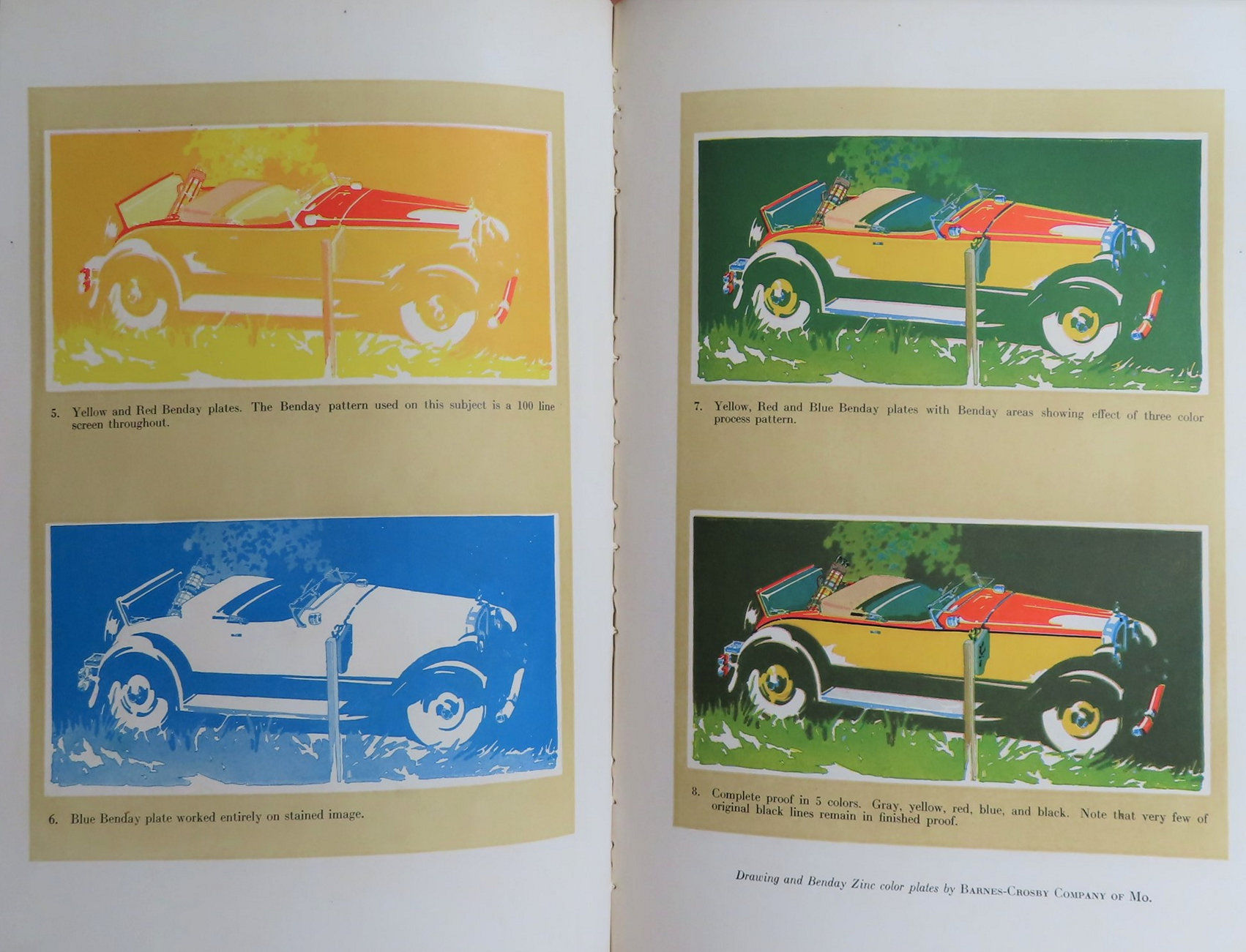The image depicts an open book displaying a detailed progression of printmaking processes for a car illustration across two pages. On the left page, the top image is labeled "5" and features an old-timey car with a washed-out yellow and red hue, facing right. Below it, labeled "6," is a car image shaded predominantly in blue tones. Each image has a brief, small-text description beneath it. The right page continues the sequence with images labeled "7" and "8." The former displays a more naturalistic depiction of the car with yellow, red, and black tones, set against a green backdrop with grass. The final image, labeled "8," showcases an even more realistic rendition of the car with a detailed background featuring greenery and some black patches. Each image is bordered in white and placed on a tan rectangular background on the white page of the book. The captions indicate a sequential build-up of colors, culminating in a completed proof using five colors: gray, yellow, red, blue, and black, illustrating the diminishing presence of original black lines as the image evolves. This layout seems to demonstrate a printmaking technique, possibly akin to linoleum cutting or screen printing.